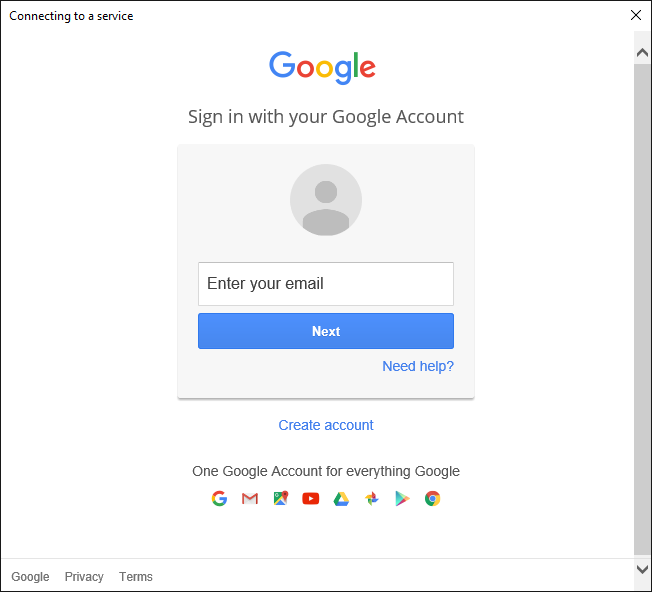**Caption:**

The image depicts a screenshot of a login page for a Google service. The window appears as a square with a white background. At the very top left corner, small black text states "Connecting to a service," and there is a close button situated in the top right corner.

Centered within the window is the prominently displayed Google logo in its traditional colors. Below the logo, gray text reads, "Sign in with your Google account." A gray box beneath the text contains a generic profile icon, which is a silhouette of a person, indicating that no user is currently logged in.

There is a white input box labeled "Enter your email," followed by a blue button with the white text "Next." To the right of this button is a link in gray text that says "Need help?".

Outside of this main login box, directly below, is another link in blue text that reads "Create account." Further down, still center-aligned, the text declares, "One Google account for everything Google." This is followed by icons representing various Google services, including Gmail, Google Maps, YouTube, Google Drive, Google Photos, Google Play, and Chrome.

At the bottom of the page is a horizontal line, beneath which it states "Google Privacy & Terms." A gray scroll bar is visible on the right side of the window, but it appears full, indicating that no additional content is available for scrolling.